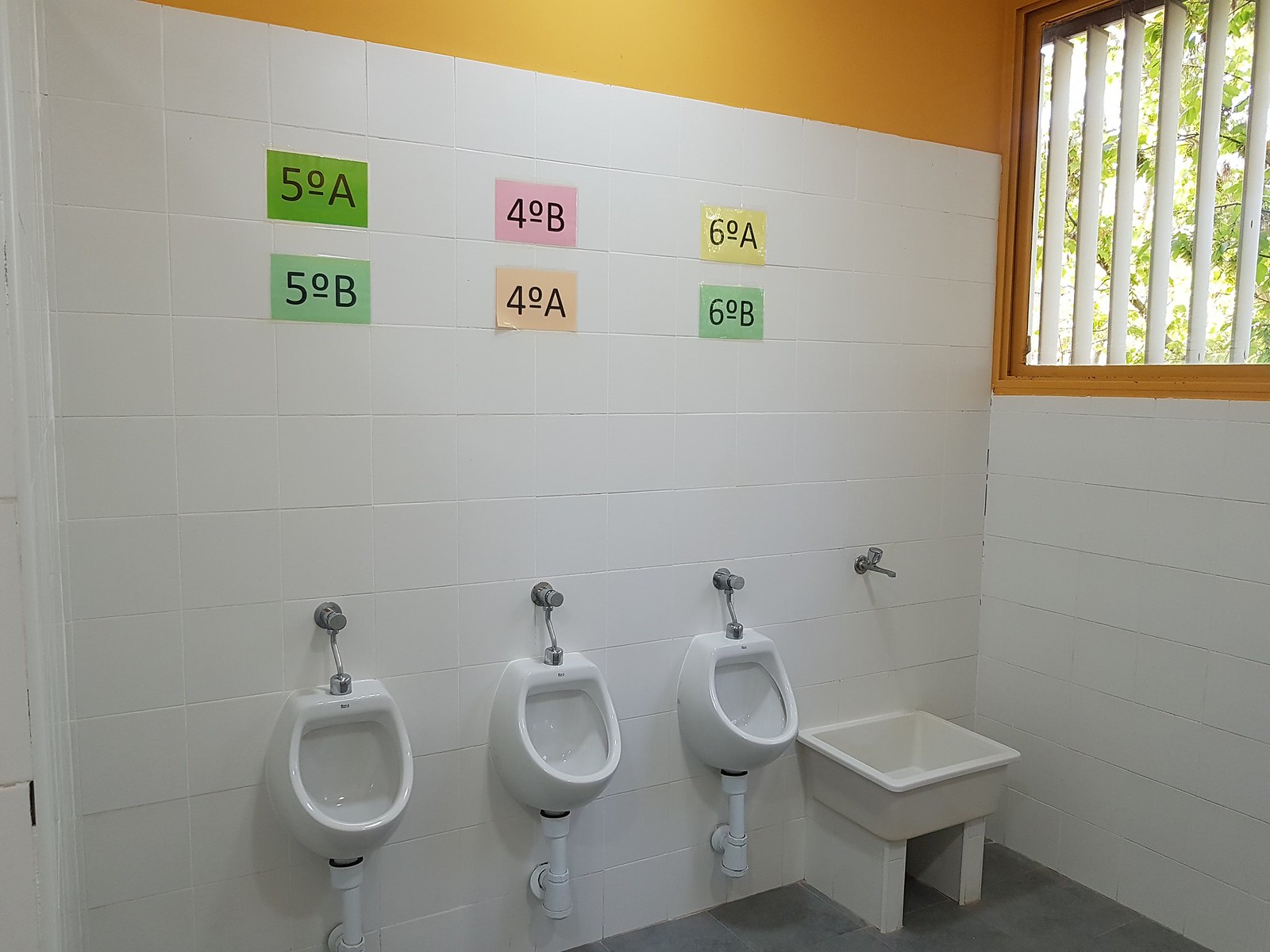The photograph captures the interior of a boys' restroom, likely in a school or a facility intended for kids. The walls are lined with white tiles, and closer to the ceiling is a bright orange-painted section. The floor is gray tile. Three small, low urinals are mounted against the wall, each with visible gray metal plumbing. To the right of the urinals is a makeshift sink—a white wash basin positioned low to the ground with a silver tap affixed to the wall above it.

Above each urinal are two signs with different numbers and letters, possibly indicating usage instructions:

- Above the first urinal: a dark green sign labeled "5-0-A" and a light green sign labeled "5-0-B".
- Above the second urinal: a pink sign labeled "4-0-B" and a peach-colored sign labeled "4-0-A".
- Above the third urinal: a yellow sign labeled "6-0-A" and a light green sign labeled "6-0-B".

In the upper right portion of the image, there's a window with open vertical blinds, revealing daylight and tree branches outside. The window itself appears to be fitted with either steel bars or further vertical blinds for added security. The restroom’s consistent white and gray color scheme, coupled with the orange trim, adds a bright and clean atmosphere to the space, punctuated by the colorful signs above the urinals.